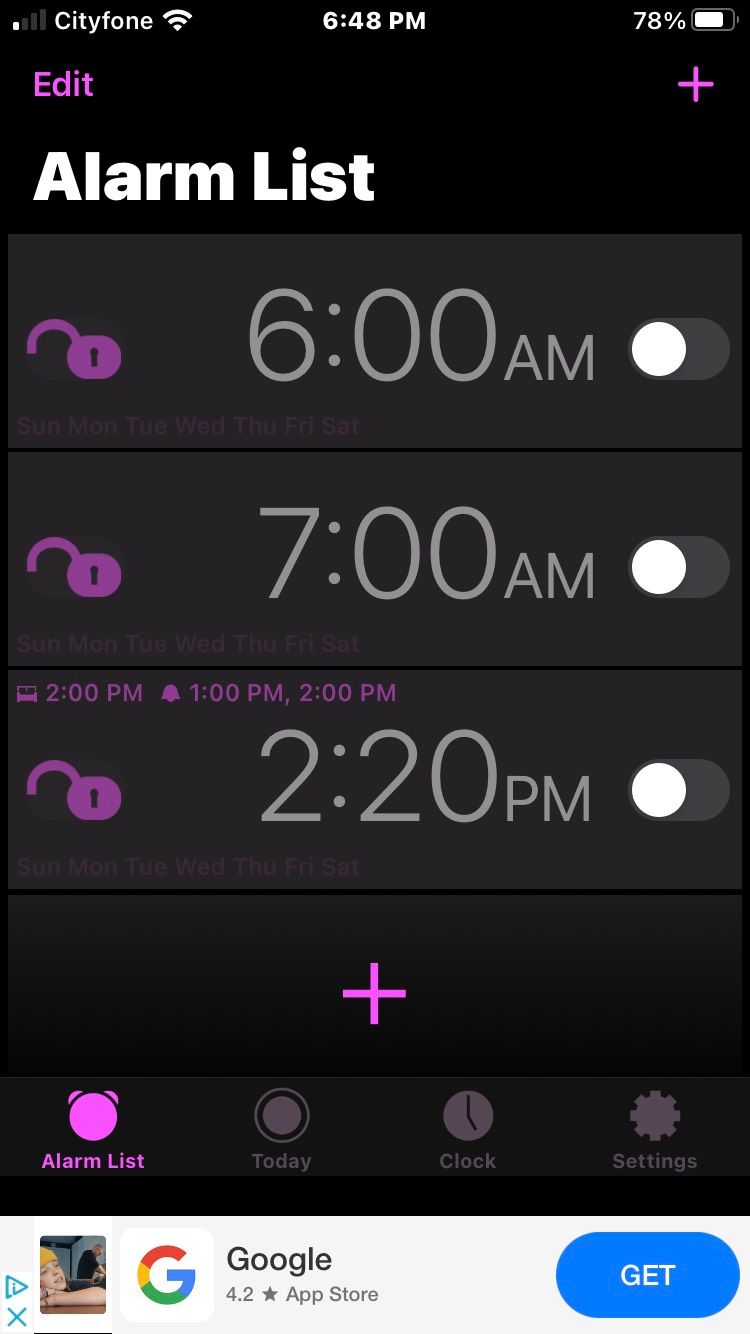This screenshot captures a phone interface featuring a mixture of black, gray, and white shades. The top two inches of the screen are black, transitioning to a light blackish-gray, with a thin black border approximately an inch from the bottom. At the very bottom is a white strip about an inch high.

In the top left corner, the internet icon appears, labeled "City Phone" in white text, followed by the Wi-Fi icon. Centrally located is the time "6:48," and on the right side, the battery percentage displays "78%" alongside a white battery icon.

Below this, "City Phone" is highlighted in purple, accompanied by an "Edit" option under the battery icon. Directly beneath it, a purple plus sign is followed by the bolded text "Alarm List." A gray tab spans the screen's width, about an inch and a half tall, featuring a series of thin gray borders dividing sections.

Each section lists alarms: the first, an unlocked purple lock icon beside "6 AM" with the toggle switched off. The second shows an unlocked lock, "7 AM," and the toggle off. The third lists "2:20 PM" next to a similar setup, with a note above stating "2 PM" and an alarm set for "1 PM," combined with a reference to calling them at "2 PM." A purple plus sign appears at the center below these entries.

Towards the bottom right, a pink alarm clock icon is labeled "Alarm List." Adjacent is a large gray circle bordered thinly, marked "Today." A clock icon indicates "Clock Settings," followed by "Settings." In the bottom left corner, an image depicts a child resting their head on a table with a man standing behind them. The Google "G" logo and "Google" text in black sits beneath it, showing a 4.2-star rating and a reference to the Apple Store. The right corner features a blue tab labeled "Get" in white.